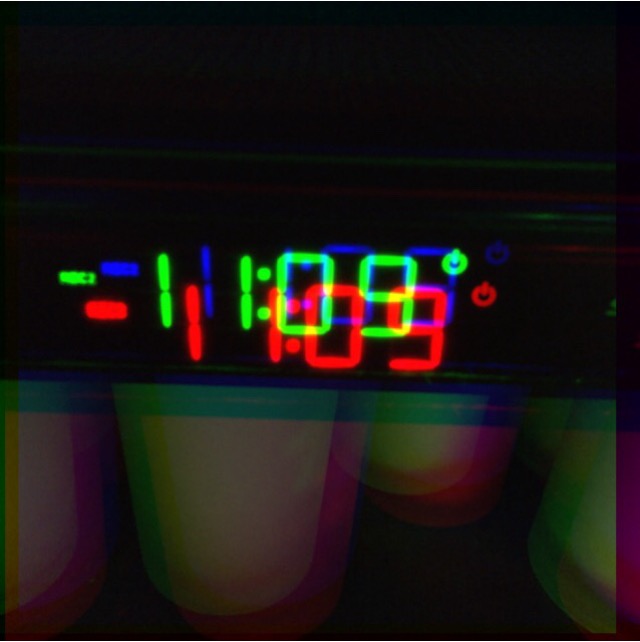The photograph displays a somewhat distorted view of an alarm clock, likely owing to a malfunction in the RGB settings of the camera. The time displayed on the clock is 11:09, depicted in both green and red, with the green digits slightly offset above and to the left of the red ones. The power symbol is also visible in this same green and red color alignment, located at the top right of the display. The image appears dark and low-quality, possibly out of focus, with significant lens flare emanating from the brightness of the LCD display, giving it a doubled, staggered appearance. There are additional unreadable texts in blue, green, and red to the left of the time display. The top half of the image is a solid black, typical of a black clock radio, while the lower part of the image has blurred elements, potentially a bed skirt or fabric, also appearing distorted with differently colored shadows due to the faulty RGB settings.